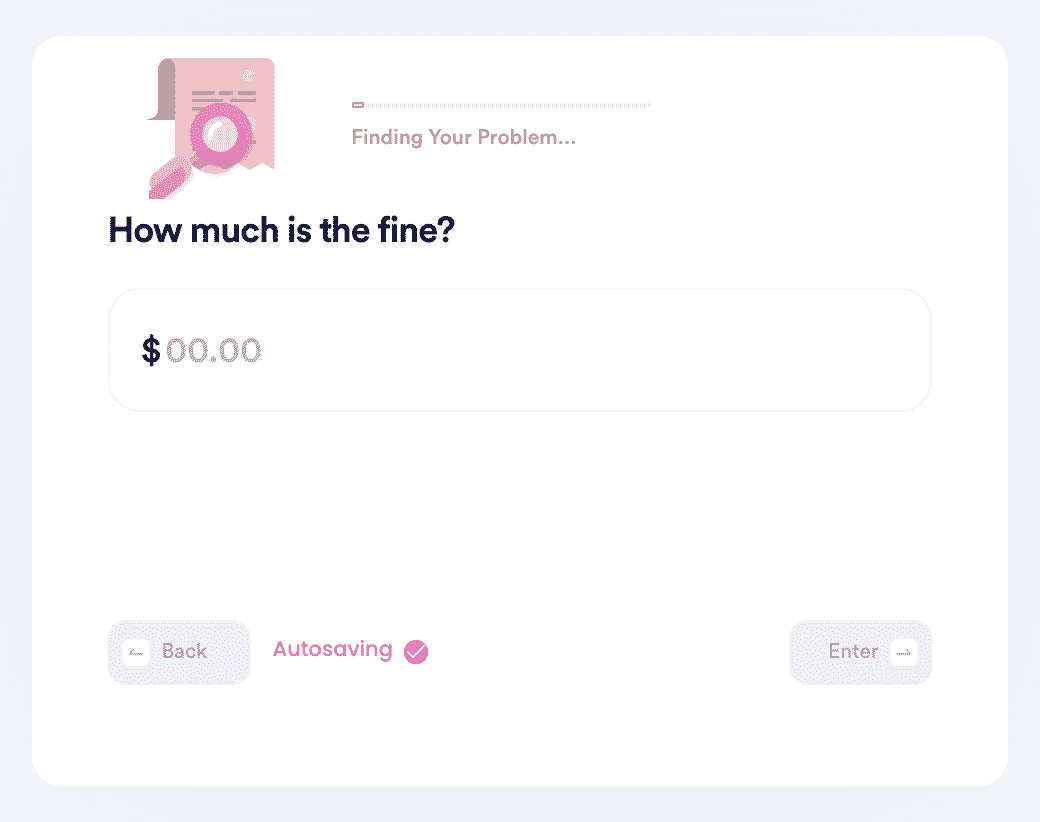The image features a light off-white background with a subtle bluish tint. Centrally positioned is a softer, inner square with rounded edges. At the top left of this square, there's a pink graph composed of lines and a small pink circle, complemented by a pink magnifying glass icon. The text "Finding Your Problem" is displayed prominently next to the graph. Beneath this, a horizontal time bar is marked to indicate a starting point.

Centered within the inner square, the bold black text reads, "How much is fine?" with options to choose from, although the amount currently shows as $0.00. Below this section, there's a light rectangular button featuring the text "Auto Saving" in purple or pink, accompanied by a square and an arrow, followed by the word "Enter."